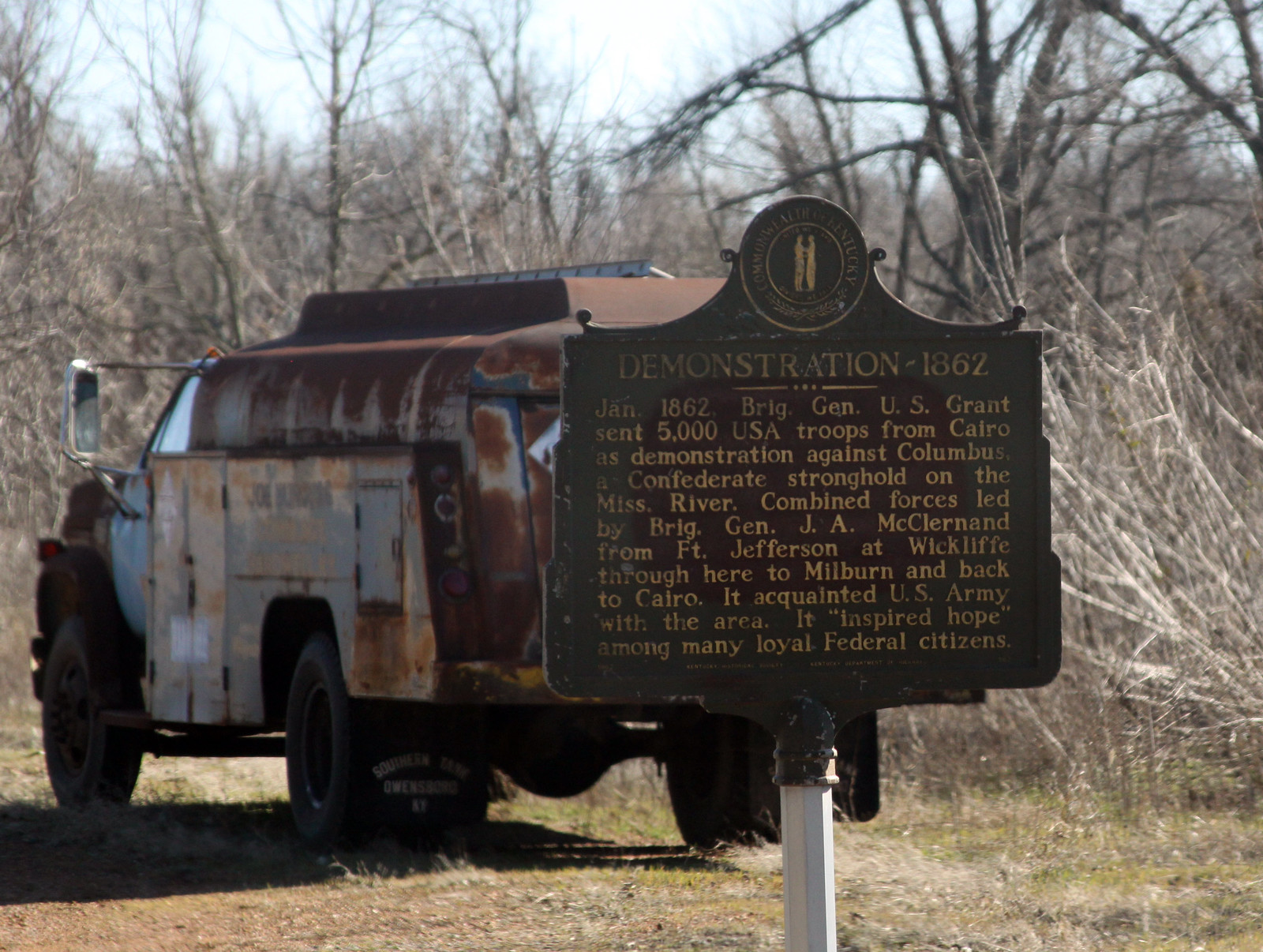This is a large square outdoor photograph featuring a historic metal sign mounted on a gray pole in the foreground. The sign is topped with a circular, brown metal emblem and is inscribed with light brown text on a dark brown background. The sign reads "Demonstration 1862" at the top and details a Civil War event where Brigadier General U.S. Grant sent 5,000 Union troops from Cairo in January 1862 as a demonstration against Columbus, a Confederate stronghold on the Mississippi River. It further explains that combined forces led by Brigadier General J.A. McLernand moved from Fort Jefferson at Wycliffe through the pictured area to Milburn and back to Cairo, familiarizing the Union Army with the region and uplifting the morale of many loyal federal citizens.

In the background, there is an old, rusted vehicle, possibly a tank or truck, characterized by gray sides interspersed with patches of brown rust. The vehicle is facing away from the viewer. Surrounding the vehicle are several leafless, bare trees, indicating a desolate or wintery setting. At the very top of the image, the sky appears slightly blurry but mostly blue, with sunlight beaming down towards the center of the scene.